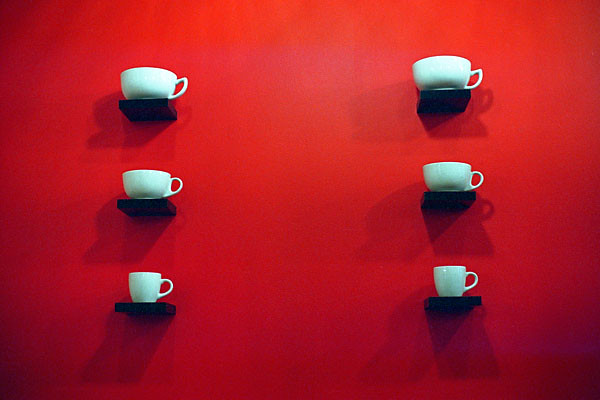This photograph features six small, square-shaped black shelves arranged in two rows of three, separated by a larger space. Mounted against a vibrant, rich cherry-red wall, each shelf holds a light teal-colored mug with a handle on one side. The mugs vary in size, with the largest ones placed on the top row, medium-sized mugs on the middle row, and the smallest mugs on the bottom row. Shadows cast by the ambient light create a gradient effect, with the top part of the image appearing lighter and the lower part darker. The light emphasizes the mugs, creating a subtle yet striking visual contrast between the teal mugs and the vivid red wall.